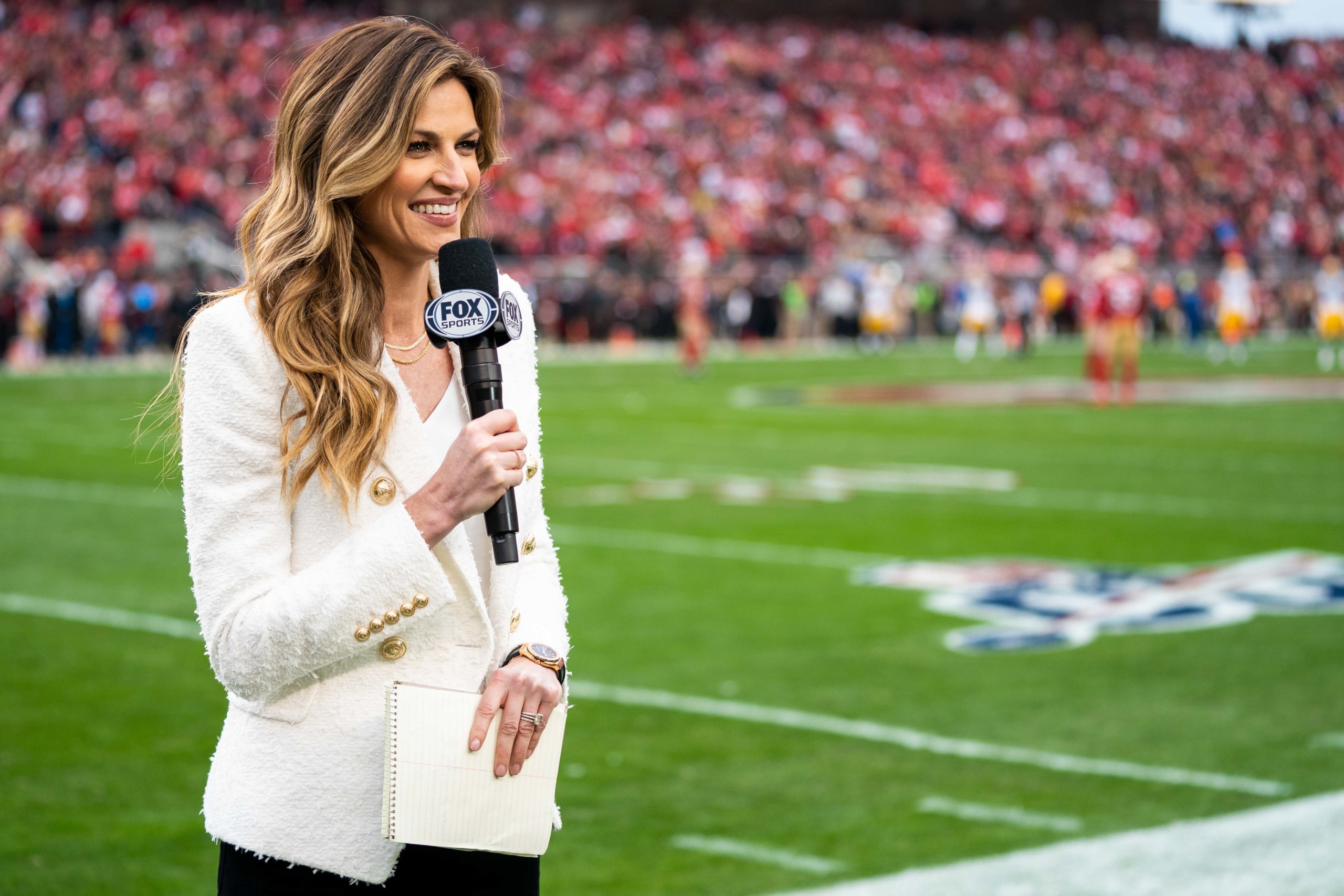The photograph captures a lively scene at an American football game, with a female reporter prominently standing on the edge of the green grassy field adorned with football markings. She is clearly identified as a sports reporter for Fox Sports, as evidenced by the large microphone she holds, emblazoned with the Fox Sports logo. The woman, who appears to be Caucasian, is smiling warmly. Her long, slightly wavy, honey-colored hair frames her face and flows over a very stylish and soft-looking white blazer decorated with distinct gold buttons on both the sleeves and the front closure. In her other hand, she holds a notebook, further indicative of her reporting role. The background, though blurred, reveals a bustling stadium full of enthusiastic fans dressed predominantly in red, suggesting a well-attended game. The woman gazes off to the right side of the image, adding an element of dynamism to the scene.